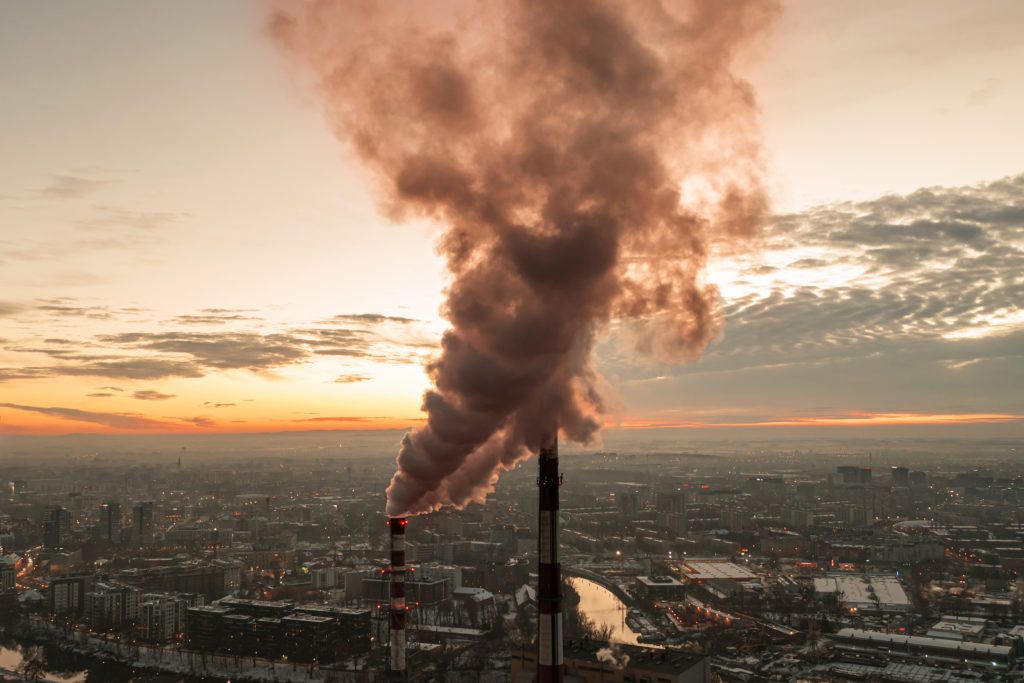This vibrant color photograph captures an expansive urban cityscape from an elevated, panoramic viewpoint, likely either from a hill or an aerial perspective. Dominating the foreground are two prominent, striped smokestacks—one black and white and the other red and white. A thick, rosy plume of smoke billows from one, almost obscuring the adjacent smokestack and occupying a significant portion of the middle frame with its pinkish, salmon-like hue. Behind this industrial foreground lies a sprawling city of high-rise apartment buildings, numbering around 24, interspersed with other large structures. A river winds its way behind the smokestacks, threading through the urban jungle and extending towards the horizon. The city stretches out extensively, fading into the distance where a mesmerizing sky transitions from pink to a striking reddish-orange along the horizon, suggesting the photo was taken either at sunset or sunrise. Wisps of clouds are visible, adding to the dramatic effect of the sky over this vast, bustling metropolis.